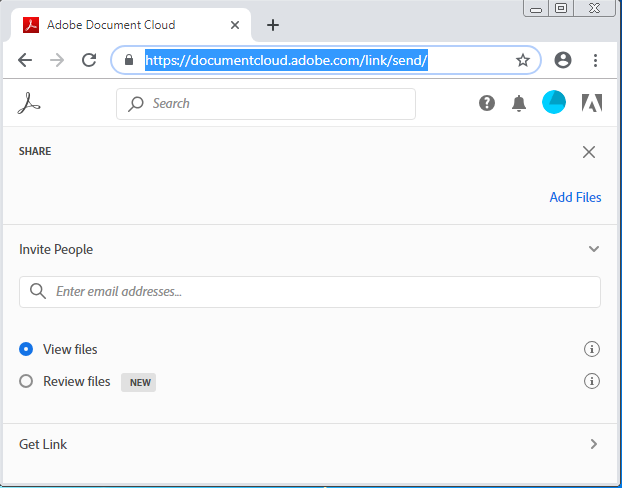**Screenshot from Adobe Document Cloud Interface**

The image is a screenshot taken from Adobe Document Cloud’s web interface, featuring a predominantly white and blue color scheme with accents of black and red. At the top left of the screenshot, the Adobe logo in red is prominently displayed next to the text "Adobe Document Cloud." 

In the upper right corner, the typical window management icons are visible: an X for closing the window, a square for maximizing it, and a dash for minimizing it. A website URL is displayed in the address bar, reading: `https://documentcloud.adobe.com/link/send/`.

Beneath the URL bar is a secondary search bar labeled "Search" with an accompanying search icon. To the right of this bar, there are several icons: a question mark for help, a bell for notifications, and two triangle icons which likely serve as navigation or alert indicators.

The interface also features an action bar with options such as "Share," an X button, and an "Add Files" button highlighted in blue. Below this bar, there is a section to invite people, displayed as a long rectangular box with the placeholder text "Enter email addresses."

Further down the interface are two options labeled "View files" and "Review files." The "View files" option is currently selected, as indicated by a blue-filled circle next to it. Both options include an information icon ("i" in a circle) at the end of their respective labels.

At the very bottom of the interface, there is a prominent "Get Link" button.

This detailed caption explains the various elements and functionality presented in the Adobe Document Cloud screenshot.